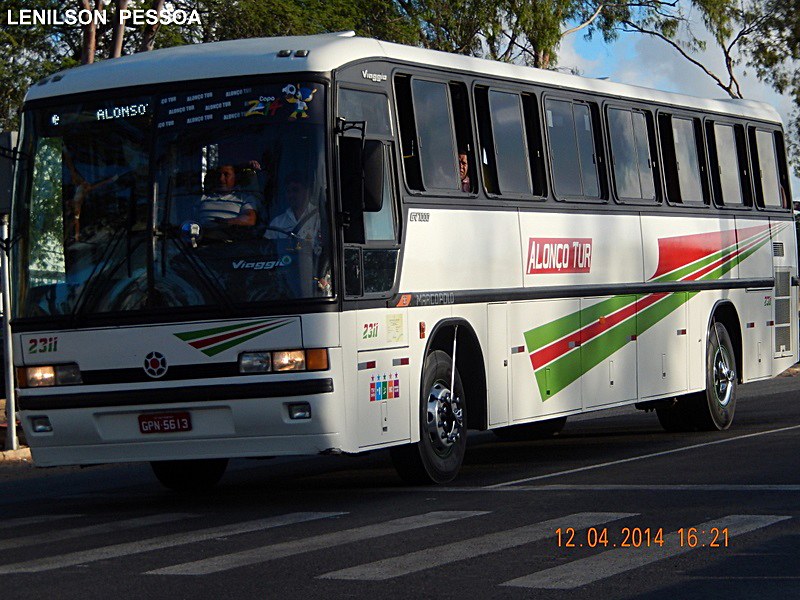The image shows a white bus with black trim and angled red and green striping on its side, identified as an "Elanco Tour" bus, displayed on a rectangular red sign with white text. The bus's headlights are on, and the timestamp in orange text at the bottom right corner reads "12.01.2014 at 16:21." Above the bus, a cloudy blue sky is visible along with some trees. The bus is stopped at a crosswalk.

Inside the bus, the driver, dressed in a white shirt, is visible through the front window. A passenger wearing a striped shirt, possibly white and blue, sits to the right of the driver. Additional passengers are visible inside. The license plate on the front of the bus reads "GPN 5613." A digital sign above the bus displays "Elanco." At the top left of the image, there is text that reads "Le Nielsen P.E.S.S.O.A. Pessoa."